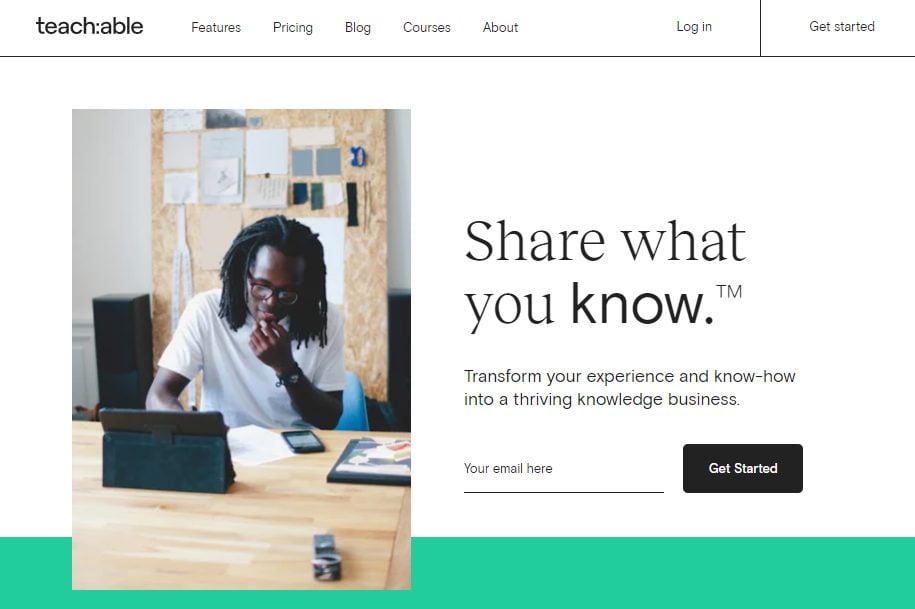The image captures the homepage of Teachable's website. At the top, the Teachable logo is prominently displayed in black text on a white background. The navigation bar includes categories such as Features, Pricing, Blog, Courses, About, and Login, along with a green "Get Started" button.

Beneath the navigation bar, there is a tagline that reads, "Share what you know. Transform your experience and know-how into a thriving knowledge-based business." An email field is provided for visitors to enter their email addresses, accompanied by a black "Get Started" button. 

Below this section, an image features a person seated at a wooden desk, engaging with a tablet. They surrounded by a smartphone and a piece of paper, are writing. In the background, a pinboard displays various pieces of paper, adding a personal touch to the workspace setting.

The majority of the webpage maintains a clean design with a white background and black text. At the bottom of the page, a green bar adds a pop of color, standing out against the otherwise monochromatic theme, creating a visually appealing contrast.